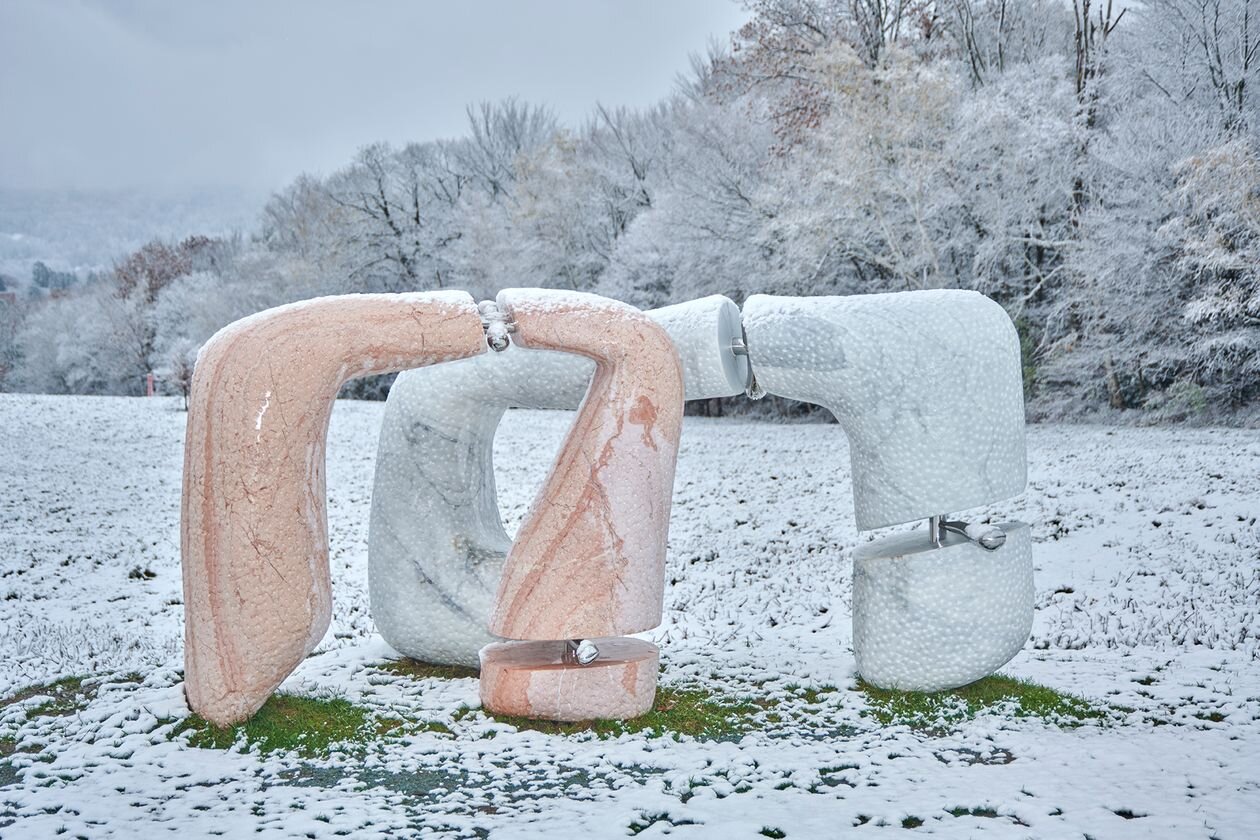In the foreground of the image, two organic, H-shaped sculptures prominently rest on a grass field lightly dusted with snow. Each sculpture consists of two interconnected, rounded shapes featuring a pebbly, stucco-like texture with variations of pink, resembling marble. The sculptures are partially overlapping, with the pink one slightly to the left, and a white one positioned behind it to the right. Both pieces have their rounded corners interrupted only where the metal connections join the separate shapes. In the background, a dense array of trees covered lightly in snow extends across the right side of the image, merging into a gray sky in the upper left corner. The overall scene combines the elements of snow-clad, lightly dusted nature with the intriguing textures and shapes of the sculptures, creating a captivating winter landscape.